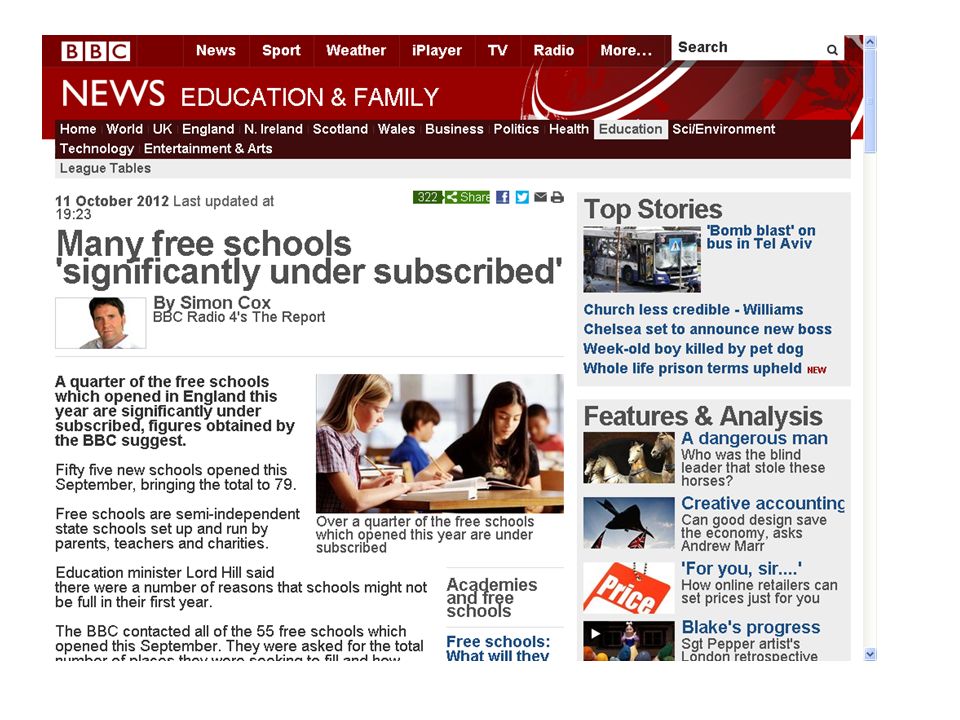Screenshot of a BBC News webpage displayed against a white background. The top navigation bar includes menu options such as "BBC," "News," "Sport," "Weather," "iPlayer," "TV," "Radio," and "More," accompanied by a search bar with a magnifying glass icon. The secondary navigation menu lists categories like "News," "Education," "Family," "Home," "World," "UK," with subcategories "England," "Northern Ireland," "Scotland," and "Wales," followed by "Business," "Politics," "Health," "Education" (highlighted in white), "Science & Environment," "Technology," "Entertainment & Arts."

The featured article is titled "Many Free Schools Significantly Undersubscribed" by Simon Cox. The article, sourced from BBC Radio 4's "The Report," indicates that a quarter of the free schools, which opened in England this year, are significantly undersubscribed. BBC-obtained figures reveal that out of the 55 new schools opened this September, bringing the total to 79, a significant number have failed to attract sufficient student enrolment. Free schools, described as semi-independent state schools, are initiated and managed by parents, teachers, and charitable organizations. A statement from Education Minister Laura Hill is featured at the end of the snippet. The update timestamp indicates the article was last modified on 11 October 2012 at 19:23. The page also features navigation links to "League Tables" and mentions various categories in smaller font under the main content.